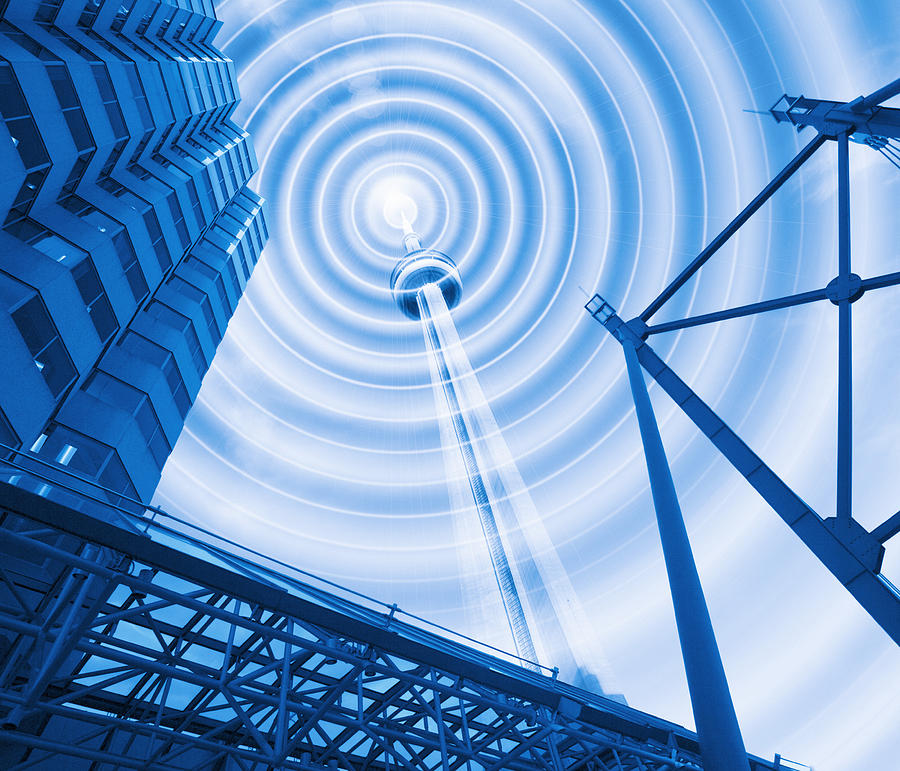This digital artwork portrays a futuristic cityscape rendered exclusively in varying shades of whites and blues. At the center of the composition stands a towering radio antenna, characterized by a transparent white elevator shaft leading up to the pinnacle of the structure. From the tip of the tower, a series of concentric white rings emanate, representing radio waves being broadcast. To the left of the tower, there's a sleek, modern building, and in the bottom-left corner, an intricate scaffolding structure can be seen, likely supporting a metallic overpass. On the right side of the image, additional metallic constructs suggest the presence of a bridge or elevated pathway. The entire scene is viewed from a ground-level perspective, evoking a sense of awe and grandeur as the viewer gazes upward at the impressive, futuristic skyline above.